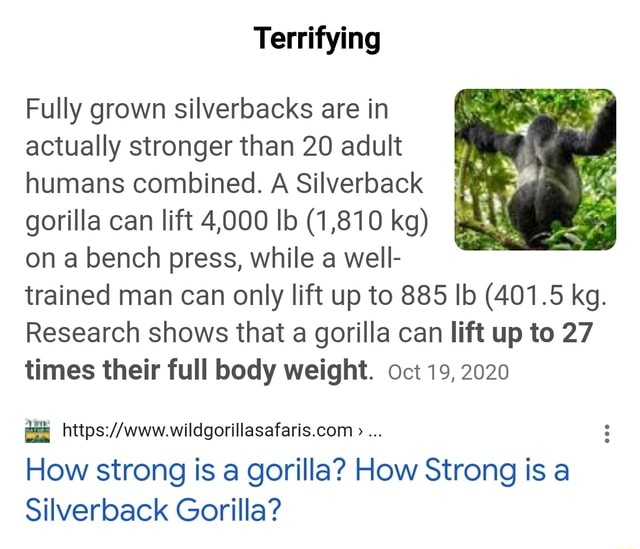A cropped screenshot of a Google search result prominently featuring the bold heading "Terrifying" at the top center. Below this, on the left side, is a description highlighted in yellow that states, "Research shows that a gorilla can lift up to 27 times their full body weight." Adjacent to the description, on the right, is a square thumbnail image displaying the back of a silverback gorilla. At the bottom of the excerpt, there's a hyperlink in large blue font reading "How strong is a gorilla? How strong is a silverback gorilla?", which, when clicked, directs users to the source website. Partially visible at the top right of the link are three dots indicating additional options, slightly cut off from view. The publication date of the information is located at the bottom right.